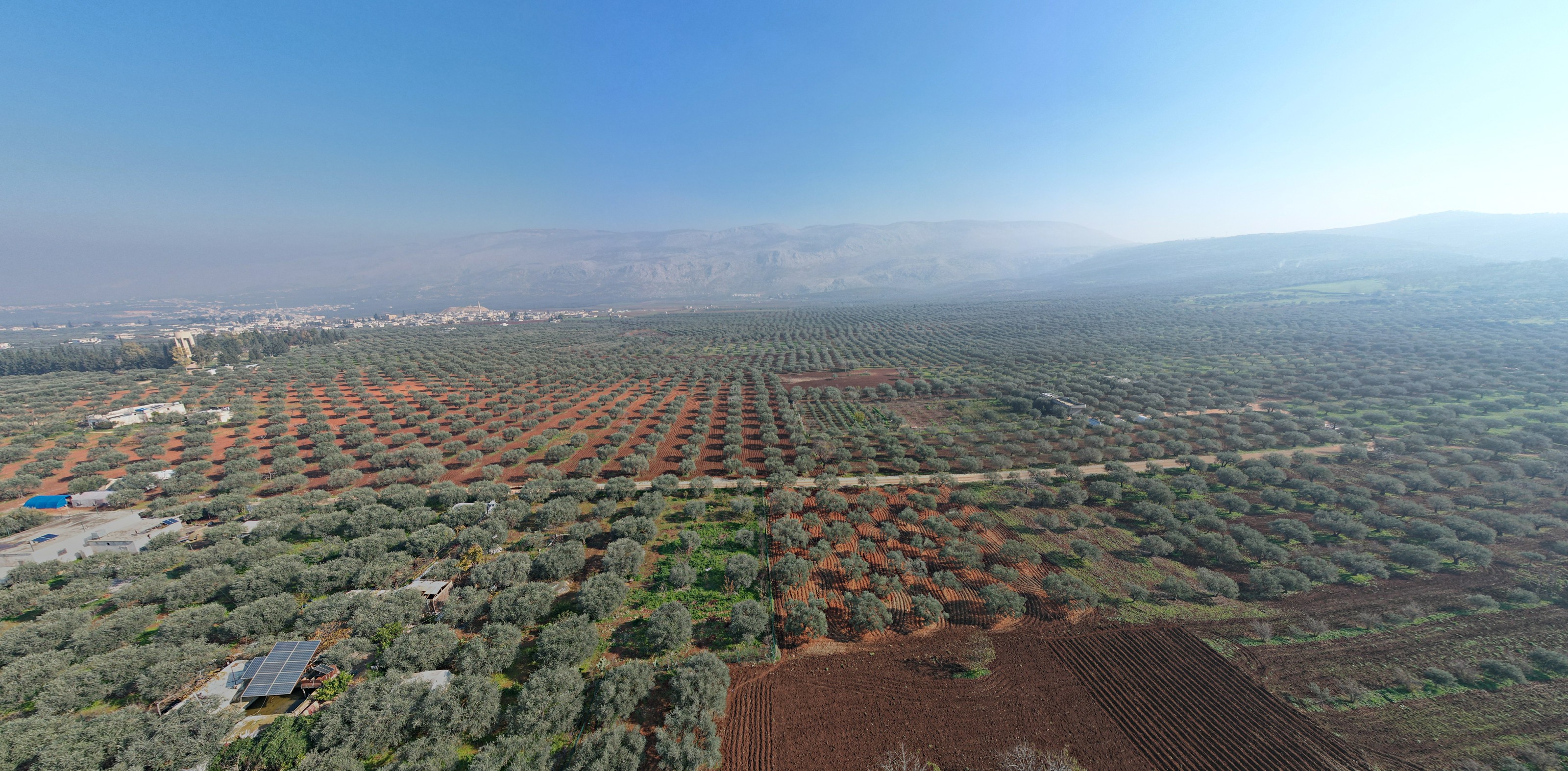This aerial image captures a detailed and organized landscape. At the top, the sky transitions from a dark blue on the left to a bright, almost white-green hue, creating a gradient effect. Below the sky, grayish mountains or hills form the backdrop. The land is divided into multiple square sections filled with rows of deliberately planted trees, suggesting tree farms. The soil beneath the trees varies in color, adding contrast between green, brown, and orange plots. The lower left-hand corner features a small black solar panel near some buildings, while the lower middle to right side of the image shows bare brown land. The consistent rows of green trees dominate the landscape, highlighting the organized agricultural layout. Further details show hints of a city in the corner, completing this richly detailed outdoor scene.